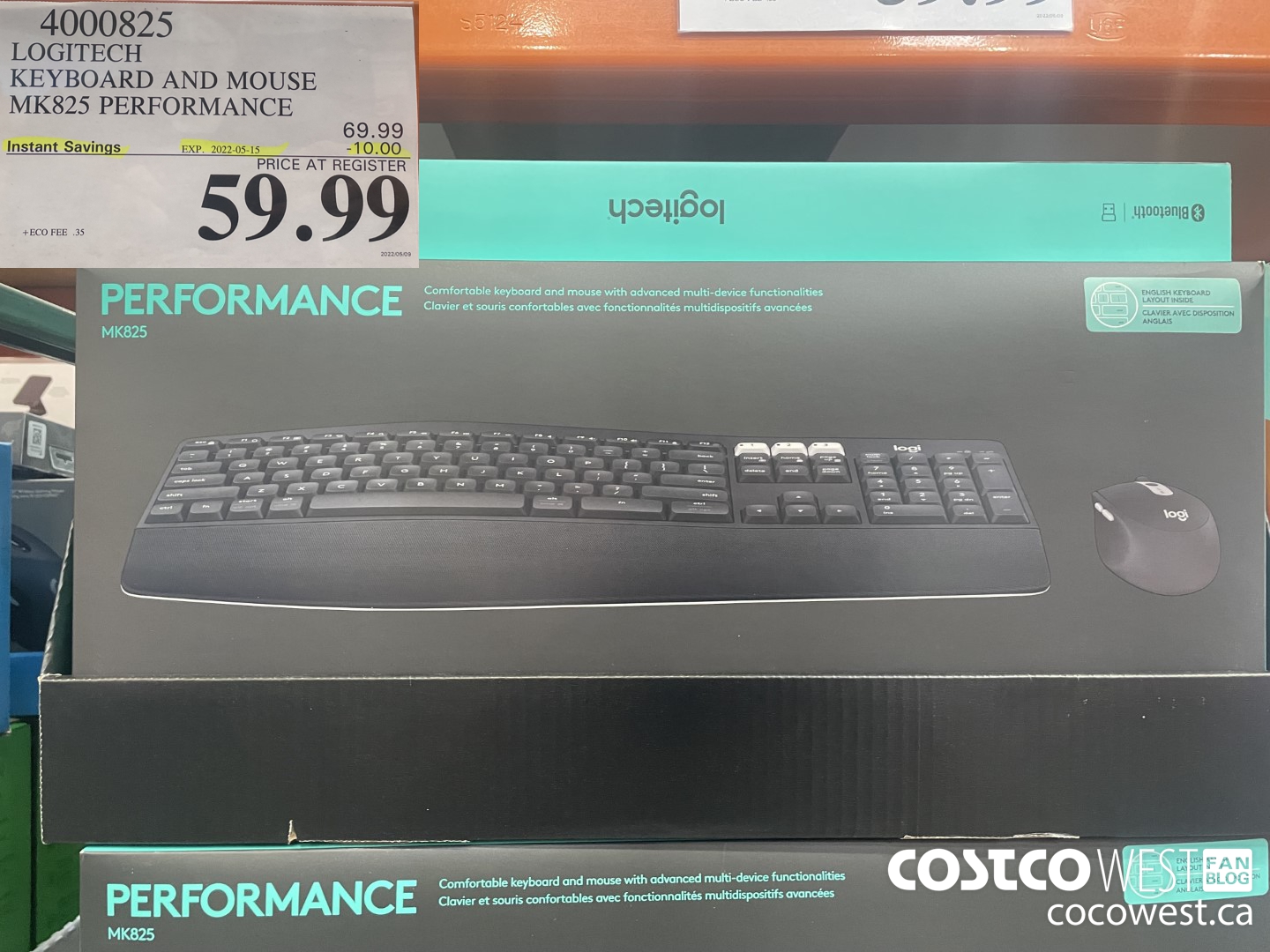The photograph captures a close-up of a retail shelf inside a store, prominently featuring a boxed set of a keyboard and mouse. The box is dark gray, emblazoned with "Performance" in turquoise lettering at the top, and below it, the model number "MK825." The package promises a "comfortable keyboard and mouse with advanced multi-device functionalities," with the identical information translated into French: "Clavier et souris confortables avec fonctionnalités multi-disposifiées avancées."

The focal point of the box is an image displaying a dark gray keyboard paired with a dark gray wrist rest, alongside a matching dark gray mouse. A label in the top right corner of the box informs buyers that an English keyboard layout is included, mirrored by the French phrase "Clavier avec disposition anglais."

An additional dark gray area at the bottom of the frame suggests part of another package of the same product is also visible. At the top left corner of the image, a white sign is taped to the shelf, providing discount information. This sign reads, "4000825 Logitech keyboard and mouse MK825 Performance. Instant savings expires 2022, 5-15, $10 off." The savings details are emphasized with yellow highlighter. The sign further indicates that the original price of $69.99 has been reduced to $59.99 at the register.